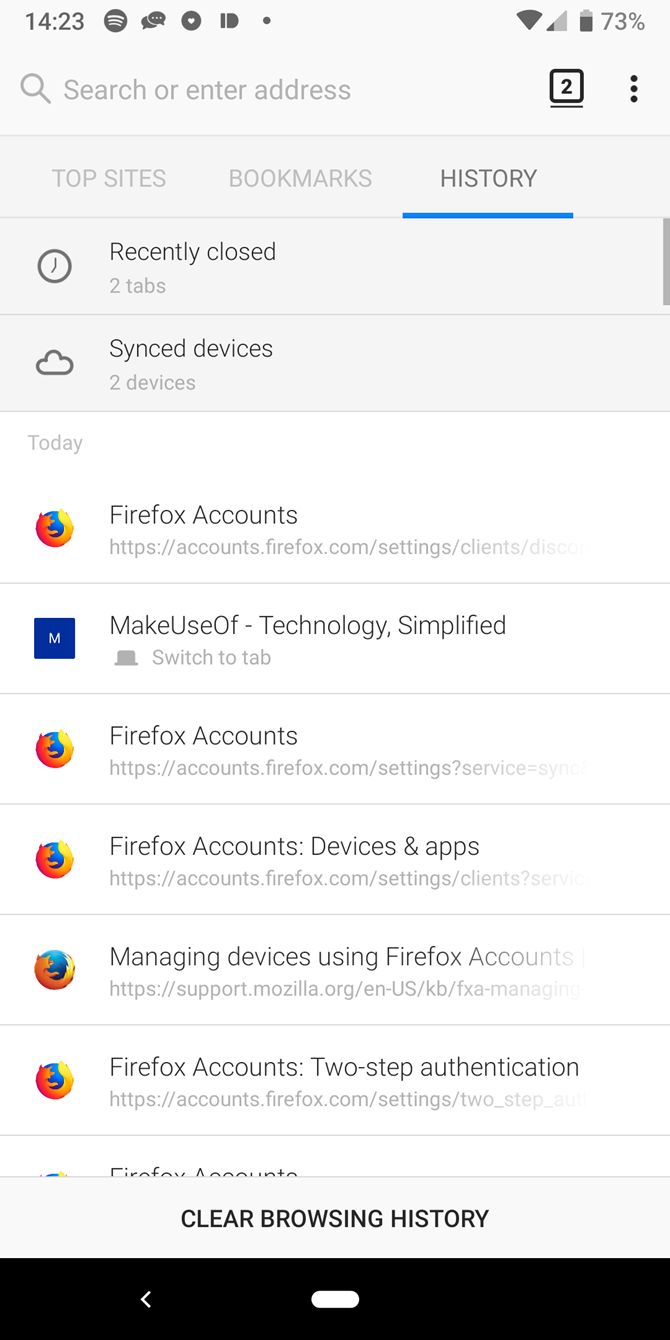Sure, here is a cleaned-up descriptive caption for the image:

---

The image showcases a screenshot of a Firefox account settings page. At the top, there is a tab list indicating two open tabs. On the left side, under the navigation bar, several menu items are visible, including "Top List (1423)," "Spotify," "Speech Bubbles," "Circle," and "Dot". Various icons such as a magnifying glass representing search functionality and gray Wi-Fi signal symbols indicating a 73% strength are also present.

The main content of the page shows options related to managing a Firefox account. There are headings and sections labeled as "Bookmarks," "History," "Closed Tabs," and "Sync Devices," showing details such as the number of synced devices (two devices as of today). 

Additionally, there are links to further settings and functionalities including "Firefox Accounts" and "Managing Devices Using Firefox Accounts." There is also a section for enabling "Two-Step Authentication" for added security.

At the bottom, the page features action buttons such as "Clear Browsing History." The navigation includes a back arrow on a black bar, followed by a white oval icon, and another black bar at the bottom.

The URL visible in the address bar is "https://accounts.firefox.com/settings/clients," indicating that the user is in the Firefox account management section.